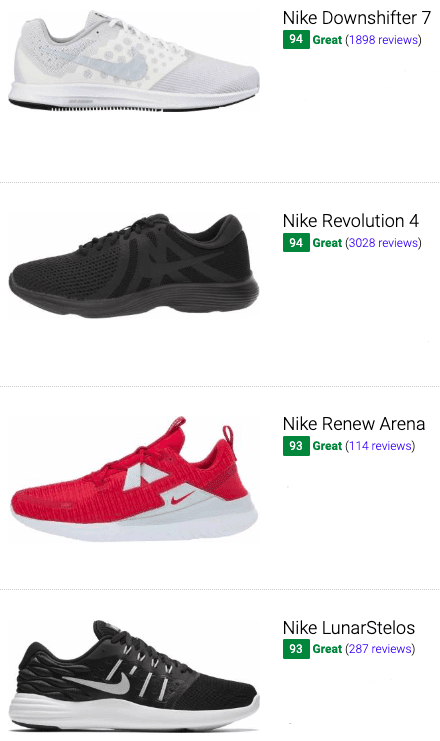The image appears to be a sales page for a website, showcasing four Nike shoes, each with detailed information about their ratings and reviews.

1. **Nike Downshifter 7**: This white and gray sneaker features a 94 score based on 1,898 reviews, indicating it is highly regarded. The shoe design includes subtle dot patterns across the lacing area and prominently displays the iconic Nike swoosh. The bottom sports black treads for added durability.

2. **Nike Revolution 4**: This model is primarily black with lighter black trim and intricate design patterns. Like the Downshifter 7, it also has a 94 score but with a higher number of reviews at 3,000. The shoe includes the signature Nike swoosh and features a higher tread pattern, offering additional traction.

3. **Nike Renew Arena**: Sporting a bold red color with white trim and a smaller Nike swoosh, this shoe is designed with a higher heel, ideal for a rocking motion while walking. It has a score of 93 from 114 reviews, showing solid feedback from users.

4. **Nike Lunar Stellos**: The fourth shoe in the lineup is black with white trim, exhibiting a more leather-like appearance as opposed to the fabric seen in the other models. It maintains a 93 score, though the number of reviews isn't specified.

Each shoe listed is accompanied by ratings, with two achieving a score of 94 and the other two a close 93, providing potential buyers with valuable insights to make an informed purchase.